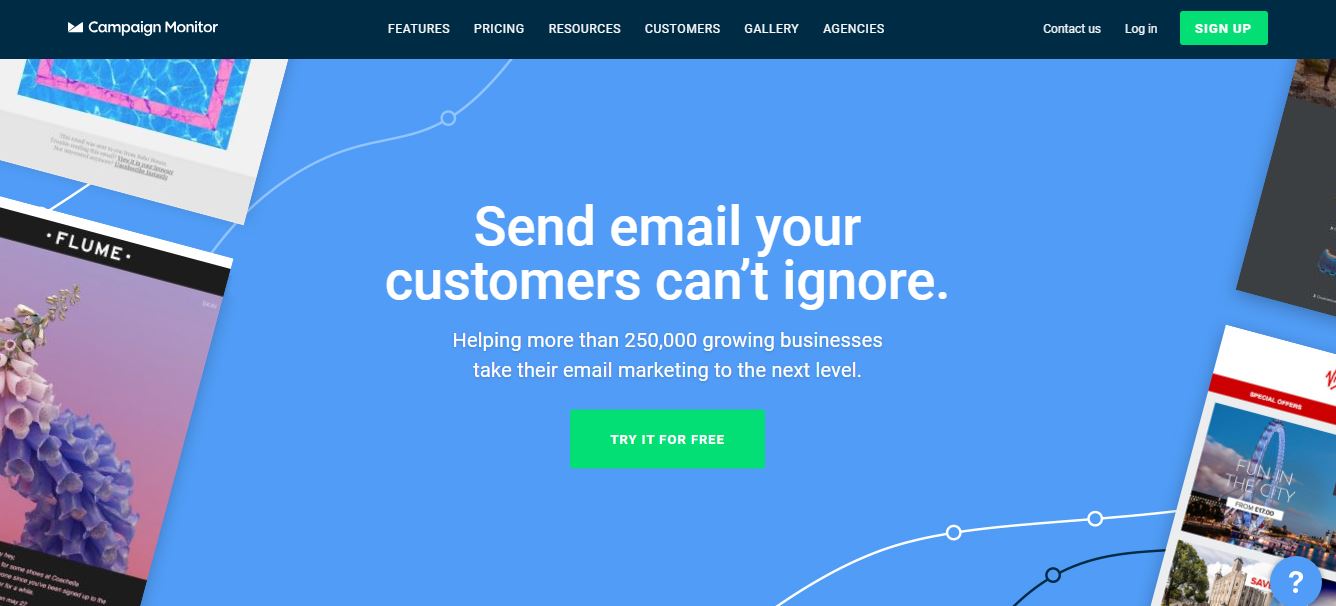This image, sourced from the Campaign Monitor website, features a user-friendly interface with navigation buttons for 'Features,' 'Pricing,' 'Resources,' 'Customers,' 'Gallery,' and 'Agencies,' along with 'Contact Us' and 'Login' options. A prominent green 'Sign Up' button invites visitors to join the platform. A bold, central message reads, "Send emails your customers can't ignore," highlighting the service's commitment to helping over 250,000 growing businesses enhance their email marketing efforts. A green 'Try it for Free' button offers a risk-free trial to potential users. The background is a serene blue, accentuated by a vibrant purple and white flower on the left and an engaging image of a cityscape to the right, featuring a ferris wheel with the tagline "Fun in the City."